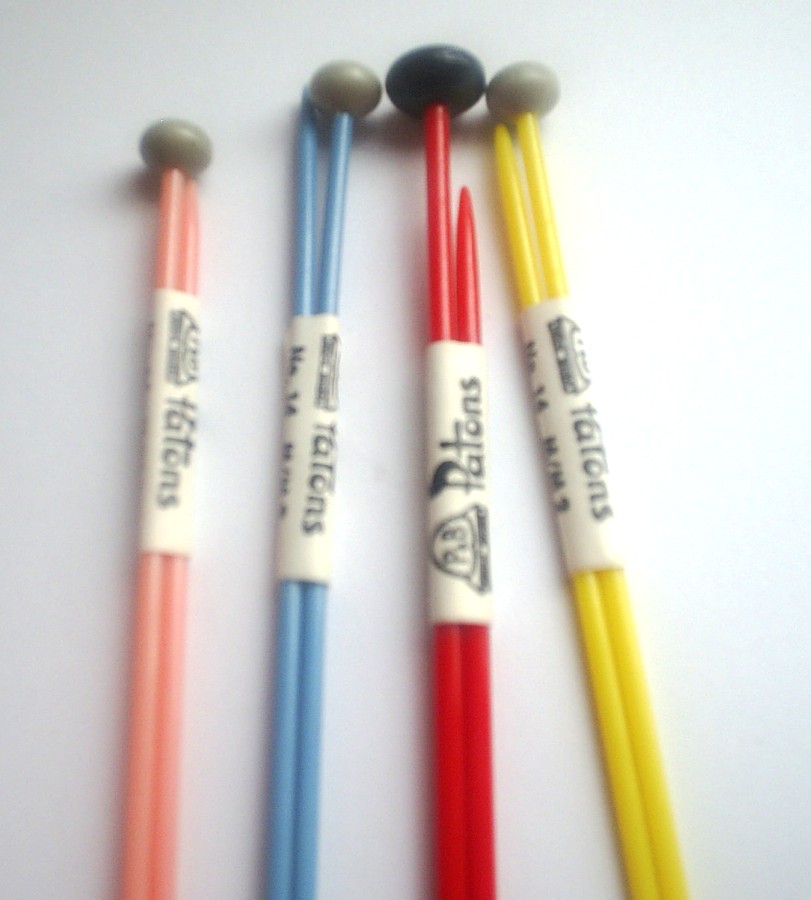On a pristine white surface, presumably a table, lie four pairs of xylophone mallets, still bundled together with their manufacturer's stickers. Each sticker is white with black text and reads "Tatons." The stickers also include a blurry, indiscernible black and white image. The four pairs are distinguished not only by the colors of their shafts but also by the colors of their rounded heads. The first, second, and fourth pairs have gray heads, while the third pair has black heads. The shafts themselves display a range of colors: the first pair boasts a pinky-peach hue, the second is sky blue, the third a medium red, and the fourth a medium yellow. Together, these colorful and well-organized mallets create a visually appealing arrangement on the white surface.